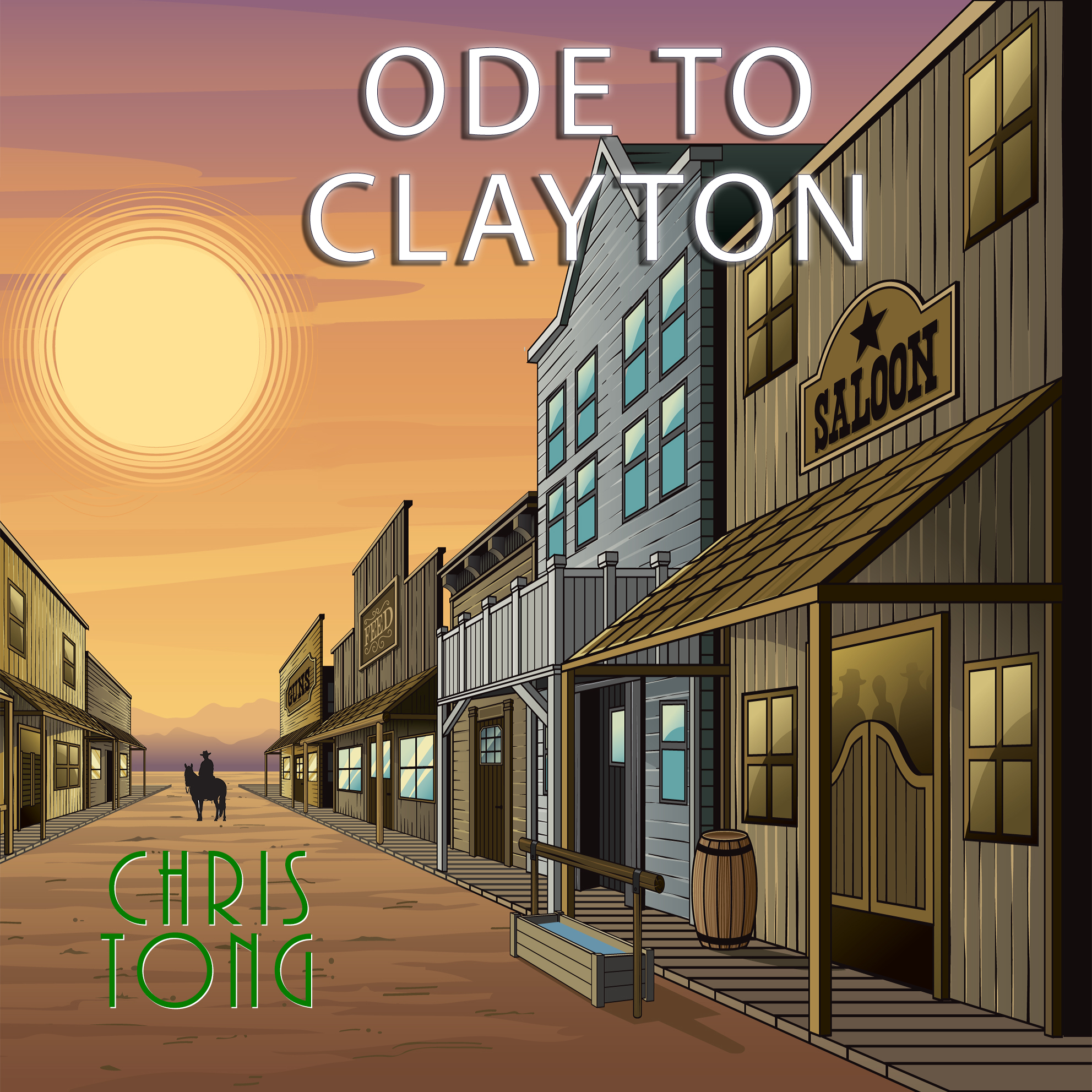The image, resembling a book cover but square in shape, depicts a meticulously detailed, computer-generated Western town under a dramatic sky painted in shades of purple, orange, and yellow. Dominating the center of the scene is a glowing, circular sun with concentric light circles. A dirt road slices through the middle of the town, leading to the silhouette of a lone cowboy on horseback. 

On the right side of the road stands a series of iconic frontier structures. The closest building, a saloon, features classic saloon doors and a sign. Shadows of people are visible behind the glass windows. In front of the saloon, a water trough and a wooden barrel underscore the town's authenticity. Adjacent to the saloon is a bluish building, followed by several more brown structures stretching into the background.

The buildings on the left side of the road are uniformly golden brown, fronted by wooden sidewalks. At the top of the image, white letters spell out "Ode to Clayton," shadowed in brown, while the bottom left corner bears the green inscription "Chris Tong."